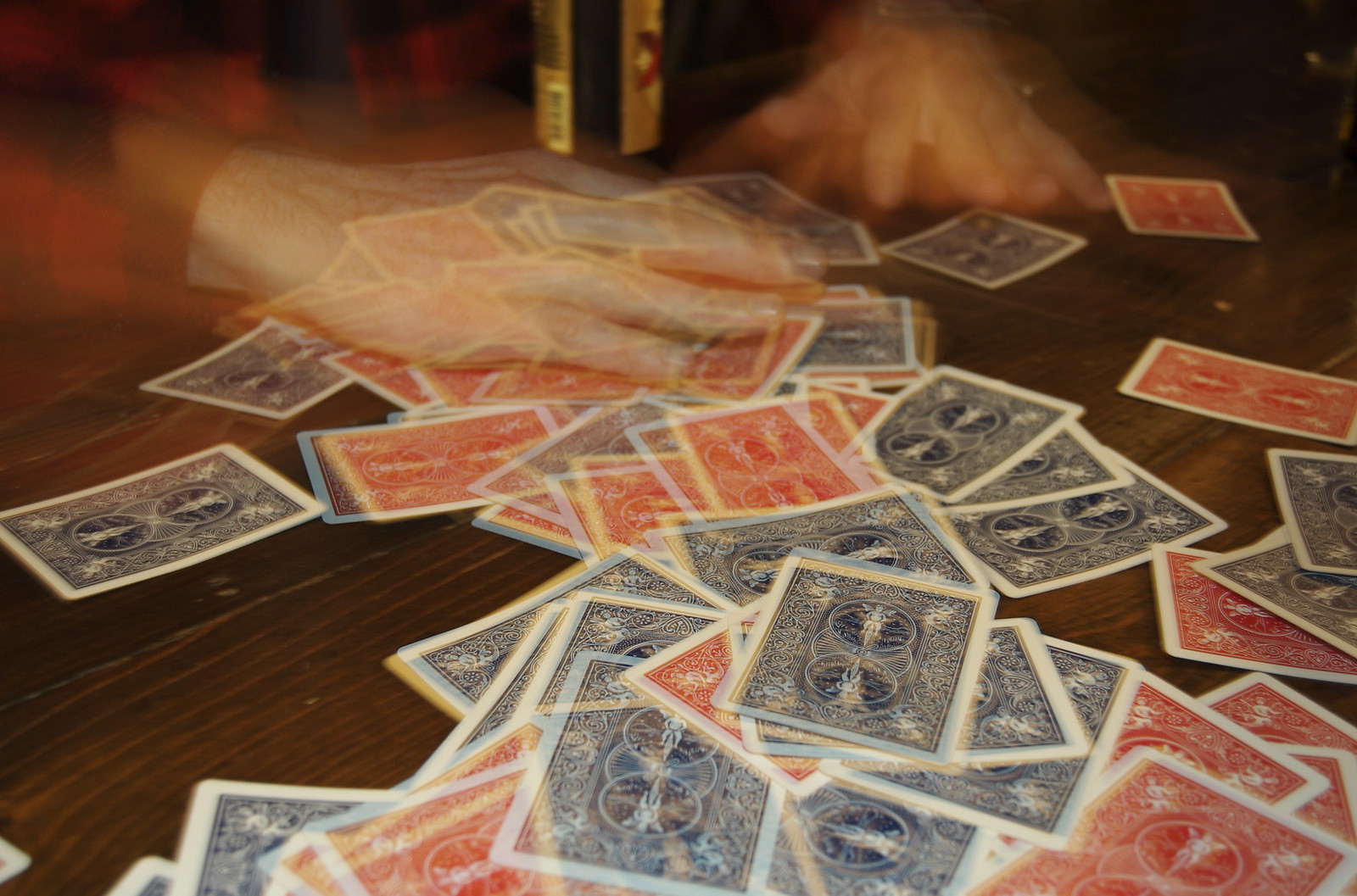In the image, two complete decks of playing cards, one red and one blue, are scattered and intermixed on a table. The cards are all facing down, with the majority of the blue cards towards the bottom of the image and a concentration of red cards near a pair of blurred hands. The hands, captured in a motion blur, appear to be rapidly shuffling the decks together, creating a ghostly effect. Most of the cards are piled haphazardly in the center of the table. The scene is dimly lit, with a hint of light emanating from the top middle portion of the image, possibly from a slightly open door, adding a mysterious ambiance to the overall dark setting.